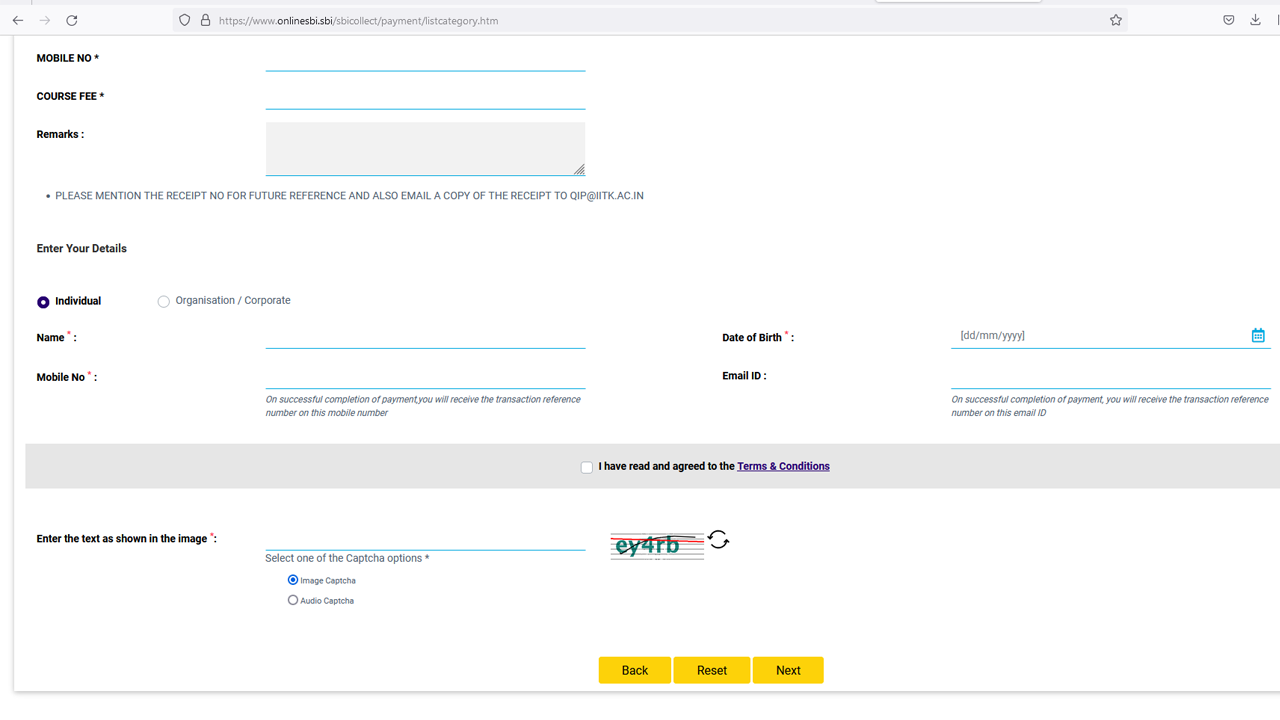**Detailed Image Caption:**

The image depicts a screenshot of a web page, which appears rather small in size. The browser’s navigation bar is visible at the top, featuring standard elements such as the back arrow, forward arrow, and refresh button. The web address in the address bar is safeguarded by a shield and lock icon, indicating a secure connection, though the exact URL is too small to be discerned. To the right of the address bar, there are icons for adding the page to favorites, downloading content, and possibly more options not entirely visible in this view.

Within the web page content, key sections are highlighted in various colors for emphasis. A mobile number is prominently displayed in bold, dark black font. Adjacent to it, a blank bar highlighted in blue catches attention. Another blank spot, labeled "Course Fee," is similarly marked in blue on the right. The "Remarks" section stands out in a blue-highlighted box, containing text that instructs users to "Please mention the receipt number for future reference" and to email a copy of the receipt.

The form on the page requires users to enter details, with "Individual" selected, indicated by a blue circle. Several mandatory fields are marked with a red asterisk: Name, Mobile Number, Date of Birth, and Email ID. At the bottom of the form, a checkbox confirms that the user has read the terms and conditions, with the "Terms and Conditions" text presented as a blue hyperlink, underscoring its importance.